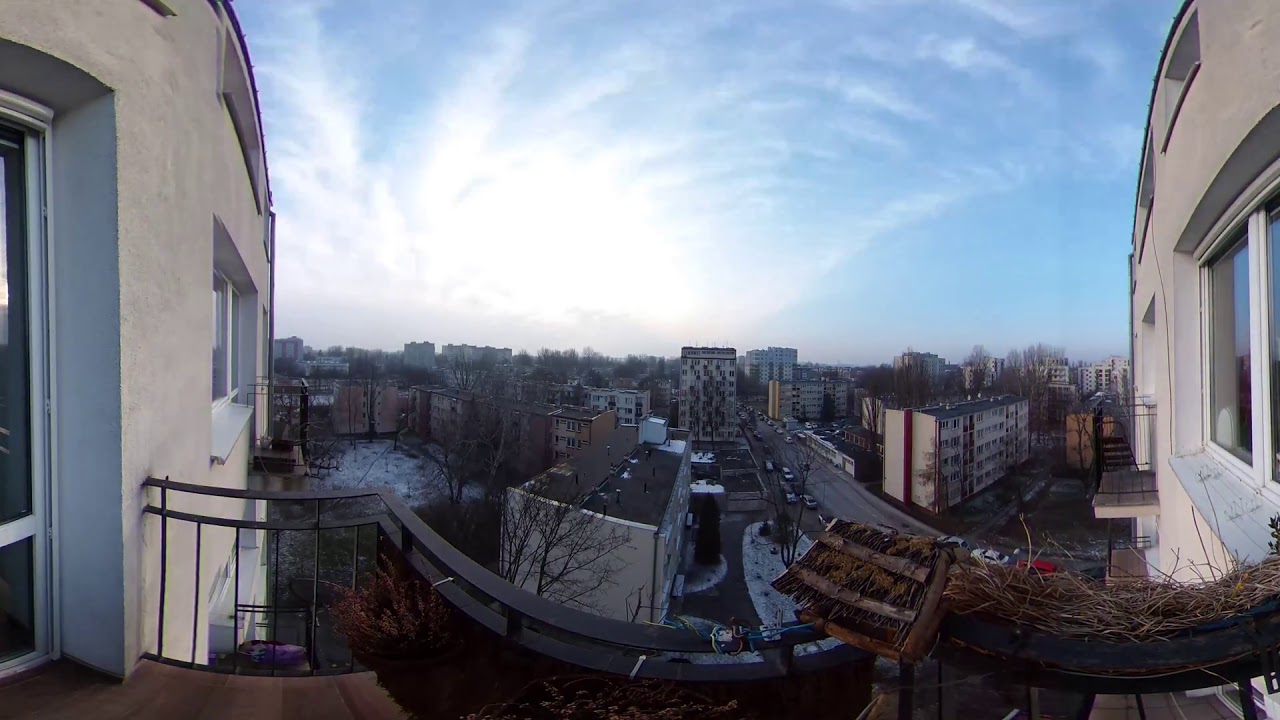This detailed urban landscape photograph is taken from the perspective of someone standing on the edge of a balcony, high up in a grayish tan cement apartment building. Looking out, the viewer is offered an expansive view of a densely built city, with multiple apartment buildings, their rooftops varying in shades of gray. The buildings on both the left and right sides of the image frame the scene, and their facades, dotted with windows and doorways, are colored in sandy or gray tones. Below, the streets bustle with parked cars, appearing tiny from this elevated vantage point. Across the way, more buildings stretch out into the distance, contributing to the densely packed urban atmosphere. A tinge of sunset hues is mirrored on the wispy clouds scattered across the blue sky, suggesting that the photo was taken towards the end of the day. The color palette includes shades of blue, gray, white, off-white, black, tan, red, yellow, orange, and purple, adding richness to the overall scene. The entire cityscape, with its mix of buildings, roads, cars, and interspersed trees, unfolds under the serene afternoon or early evening sky.